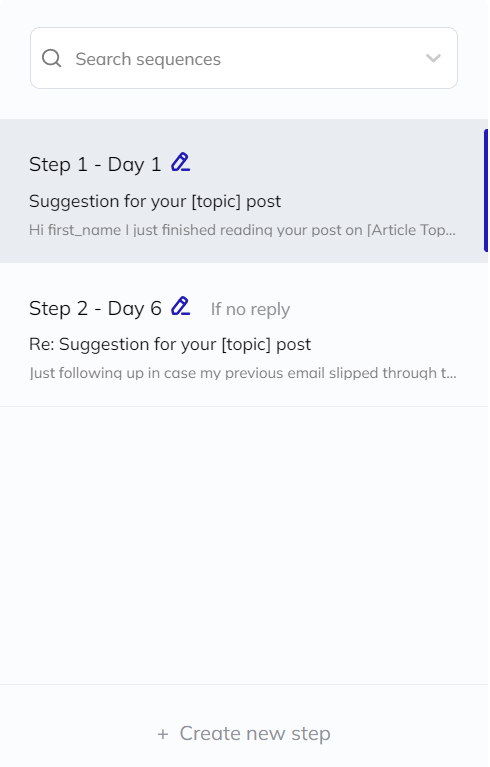This image is a portrait-mode screenshot of a web interface featuring a to-do list or a sequence of steps. The background is an off-white color throughout the image, which is organized into a single long column.

- **Top Section:** The uppermost part of the screenshot displays a search bar spanning from the upper left-hand corner to the upper right-hand corner. Within the search bar, the text "search sequences" is typed, and there is a down arrow icon on the right side of the bar, presumably for a drop-down menu.

- **First Row:** The row immediately below the search bar is highlighted in gray. It is labeled "Step 1, Day 1" and includes a pen icon on the right side, suggesting an edit function. This row contains the phrase "Suggestion for your [topic post]" where the placeholder could be a customizable topic such as "gardening post" or "work from home post." Below this, the text reads: "Hi [First Name], I just finished reading your post on [article topic]." On the far right is a vertical blue stripe, likely serving as a visual indicator or accent.

- **Second Row:** The subsequent row is labeled "Step 2, Day 6," and also has a pen icon for editing purposes. This row contains the text: "If no reply then regarding suggestion for your [topic post], just following up in case my previous email slipped through the..." This suggests a follow-up step in an email sequence. At the bottom of this row is a prompt to "Create New Step," indicating an actionable item to add more steps to the sequence.

Overall, the screenshot captures a step-by-step process for managing or automating communications, with specific placeholders for personalizing the content.